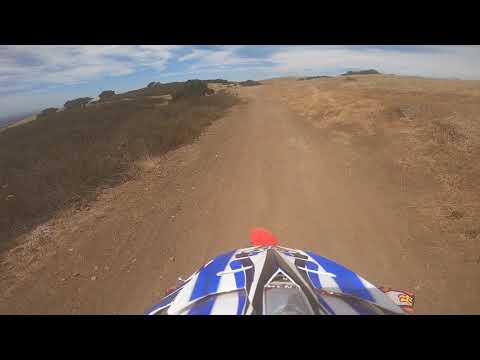The image captures the viewpoint of someone riding a dirt bike on a long, dusty trail, seemingly taken with a GoPro. The front of the vehicle, which appears to be a dirt bike, is partially visible at the bottom of the image, featuring a white base with royal blue and black accents, and a red detail near the top. There may be a number on the side of the bike. The trail stretches far into the distance, flanked by dead grass to the left and sand to the right, with small rocks scattered along the path. The setting is a barren desert or savannah, with sparse vegetation and distant dead-looking trees on the horizon. The sky is cloudy, lending the scene a somewhat overcast ambiance. There are no buildings, other vehicles, or people in sight, indicating the rider is alone in this vast, open landscape. The colors in the image include shades of brown, tan, gray, blue, green, and light blue. The overall atmosphere suggests a solitary ride through a remote, rugged terrain.